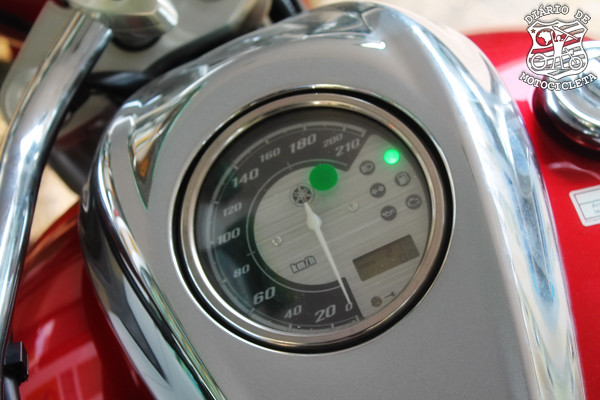In this highly detailed close-up image, we see the intricate design of a motorcycle speedometer. The speedometer is mounted on a gleaming silver metallic surface and encased in clear glass for protection. A stark white needle arcs across the instrument, designed to indicate speeds as the motorcycle accelerates. The speedometer features white numerical markings denoting speeds at intervals: 0, 20, 40, 60, 80, 100, 120, 140, 160, 180, 200, and 210. 

Adjacent to the speed marker is a section designated for indicators, with a small green light visibly illuminated. This entire setup is situated on a striking red chrome base, adding a vibrant contrast to the polished silver components. Just visible are the edges of steel handlebars, suggesting robust control and handling. 

In the extreme right corner of the image, the top of the fuel tank is partially visible, characterized by its silver finish and adorned with a distinctive symbol. There is also a phrase in a foreign language—"Dario da Motoclita"—written in white letters, accompanied by a figure of a person on a motorcycle.